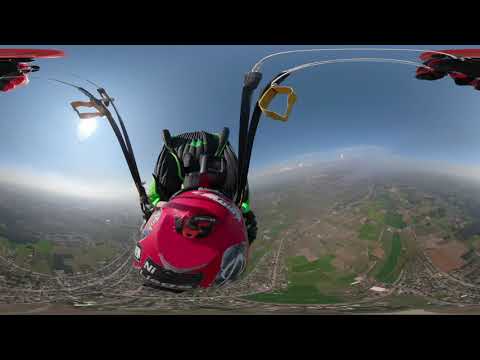This image captures a 360-degree view of a skydiver in mid-air against a backdrop of clear blue skies with a visible yellow sun on the left-hand side. Below, there is a topographical perspective showing a mix of rural and urban landscapes with roads, green patches of farmland, and scattered buildings. The main subject is the skydiver wearing a red helmet and carrying a black and green parachute bag. The parachute itself is red with black ropes extending from the top. Additional white ropes with red objects attached at their ends and yellow cufflinks are seen on either side. The scene is possibly slightly distorted, giving it a fisheye lens effect.